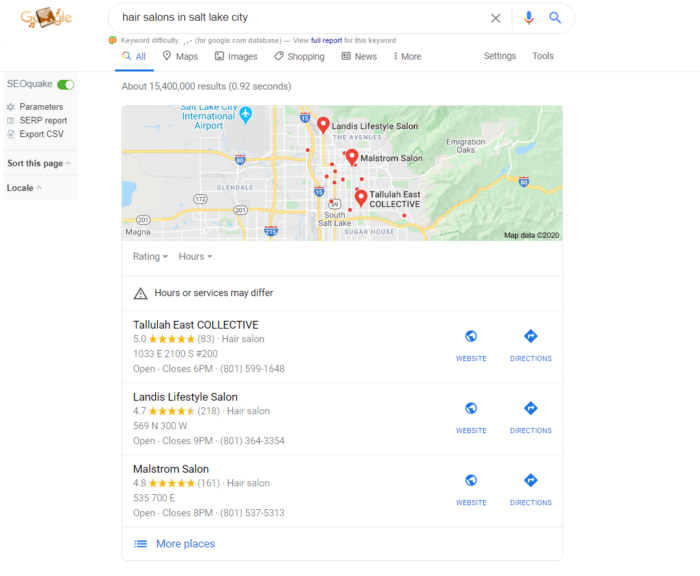The image depicts a Google search results page for hair salons in Salt Lake City. The Google logo appears at the top, although it looks somewhat different from the standard version. Below the search bar and headings, a map segment highlights part of South Salt Lake. The map features three red location markers indicating hair salons: Landis Lifestyle Salon, located above the avenue; Maelstrom Salon, positioned in a densely built-up area; and Tallulah East Collective, situated near South Salt Lake. Additionally, a blue flag with an airplane icon marks the location of Salt Lake City's international airport in the upper left corner. Beneath the map, brief descriptions of the three salons are provided.